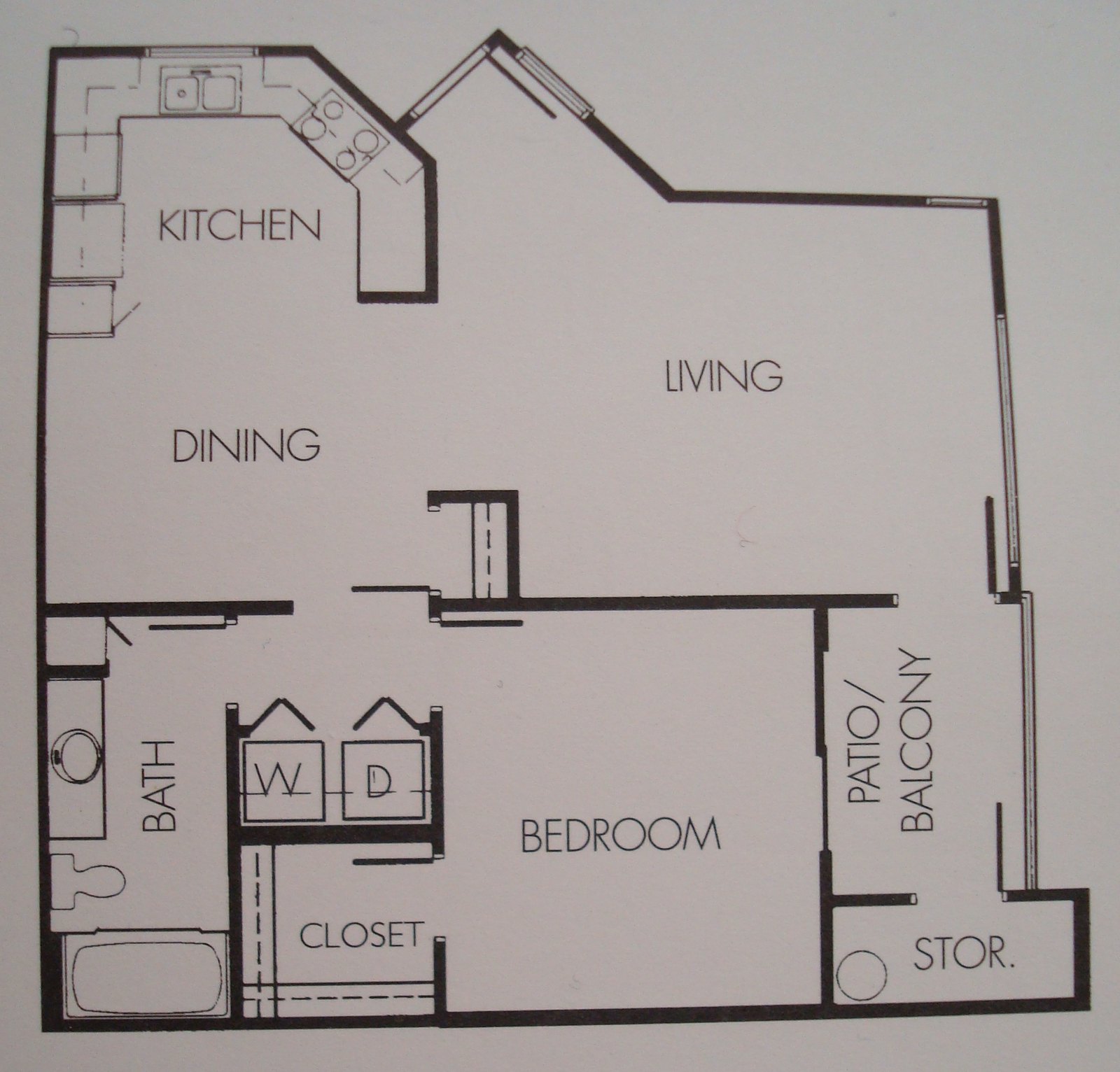A meticulously detailed, computer-generated blueprint of a house is depicted against a white background with black text and line work. This blueprint illustrates a primarily square structure. 

In the upper portion, the living room area features a distinctive pointed ceiling, drawing attention to its architectural design. The upper left corner is labeled "Kitchen," showcasing detailed elements like countertops, a stove, and a sink. Adjacent to this, the area marked "Dining" appears notably spacious and uncluttered. 

On the upper right side, the "Living" area is demarcated, leading downwards through a hallway. The lower left corner contains a "Bath" section, complete with a sink, bathtub, and toilet. Centrally located is the "Bedroom," which includes an attached closet to the left. Directly left of the bedroom is labeled "WD," indicating space for a washer and dryer, represented by two distinct rectangular shapes.

To the right of the bedroom, two separate areas are distinguished: "Patio/Balcony" and "Storage." The "Storage" room is situated in the lower right corner and intriguingly contains a circular object at its center. The blueprint offers a comprehensive and clear representation of the house's layout, meticulously detailing each room's purpose and features.